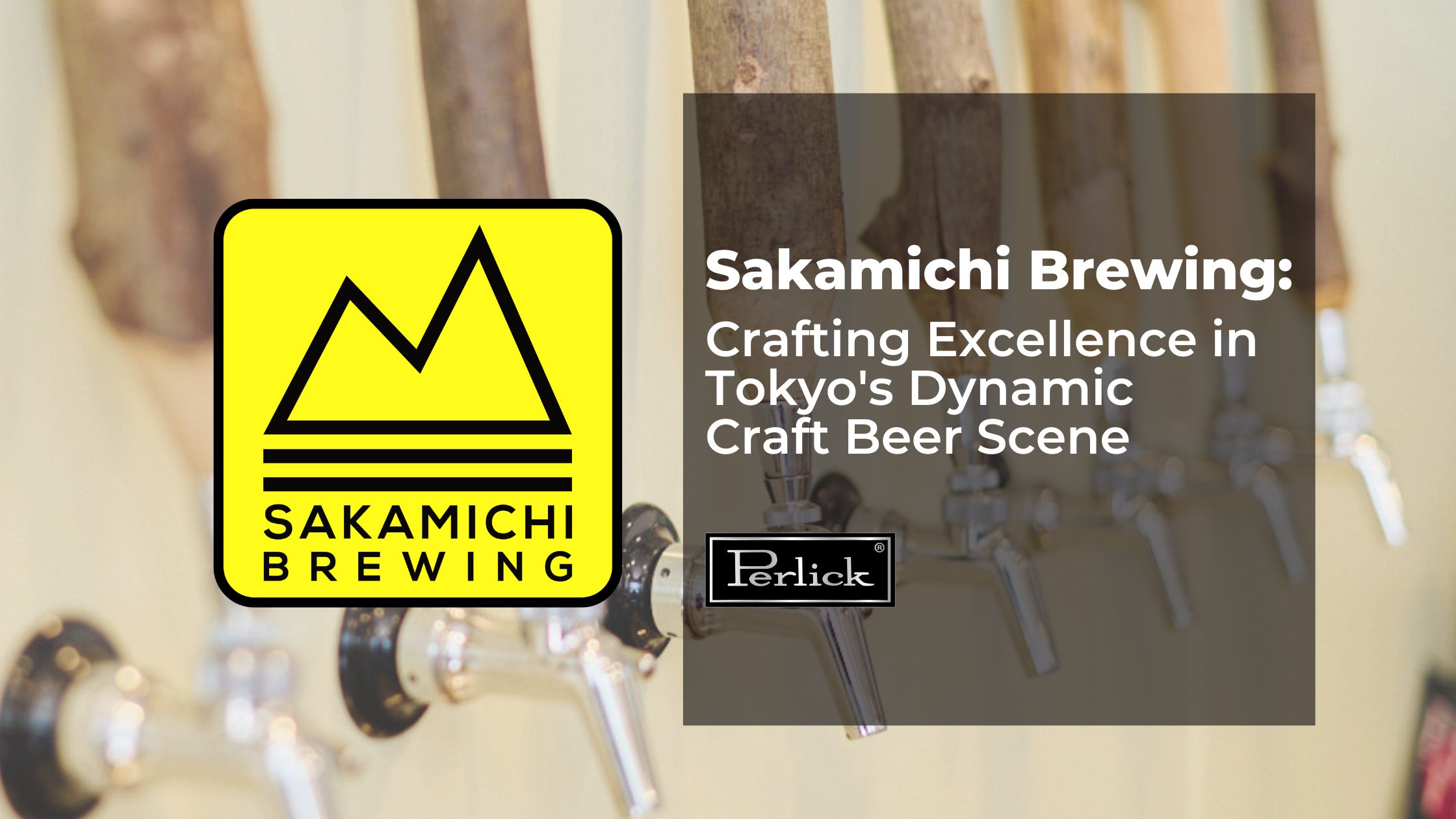This advertisement features a close-up photograph of intricately carved tree limb beer taps, each fitting seamlessly into clear valve nozzles, evoking a sense of craftsmanship and nature. Despite the proximity, the taps are slightly out of focus, directing attention to the vibrant, overlapping text overlays. Dominating the left side of the image, a yellow rectangle displays the Sakamichi Brewing logo alongside a stylized mountain graphic, symbolizing purity and adventure. Adjacent to it, a larger semi-translucent black rectangle boasts the message: "Sakamichi Brewing: Crafting Excellence in Tokyo's Dynamic Craft Beer Scene," emphasizing the brewery's dedication to quality. Beneath this, a smaller black segment marked with the brand "Perlick" in white letters underscores the premium equipment used, encapsulating the brand's commitment to delivering an exceptional brewing experience.